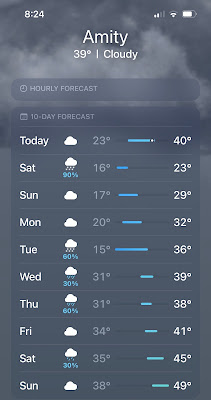This screenshot from a weather forecast app displays the weather for Amity at 8:24 AM. Currently, the temperature is 39°F and the sky is cloudy. While the image quality isn't the best, the details are still discernible. The "Hourly Forecast" section is mentioned but not visible in the screenshot. The "10-Day Forecast" section, however, is expanded and shows the following:

- **Today:** High of 40°F, Low of 23°F, Cloudy
- **Saturday:** High of 23°F, Low of 16°F, Snow, 90% precipitation chance
- **Sunday:** High of 29°F, Low of 17°F, Cloudy
- **Monday:** High of 32°F, Low of 20°F, Snow, 60% precipitation chance
- **Tuesday:** High of 36°F, Low of 15°F, Snow, 60% precipitation chance
- **Wednesday:** High of 39°F, Low of 31°F, Snow, 30% precipitation chance
- **Thursday:** High of 41°F, Low of 31°F, Snow, 30% precipitation chance
- **Friday:** High of 41°F, Low of 34°F, Snow, 30% precipitation chance
- **Saturday:** High of 45°F, Low of 35°F, Snow, 30% precipitation chance
- **Sunday:** High of 49°F, Low of 38°F, Snow, 30% precipitation chance

While the forecast provides a 10-day outlook, its accuracy may diminish with time. Currently, it emphasizes cold and snowy conditions in the coming days.